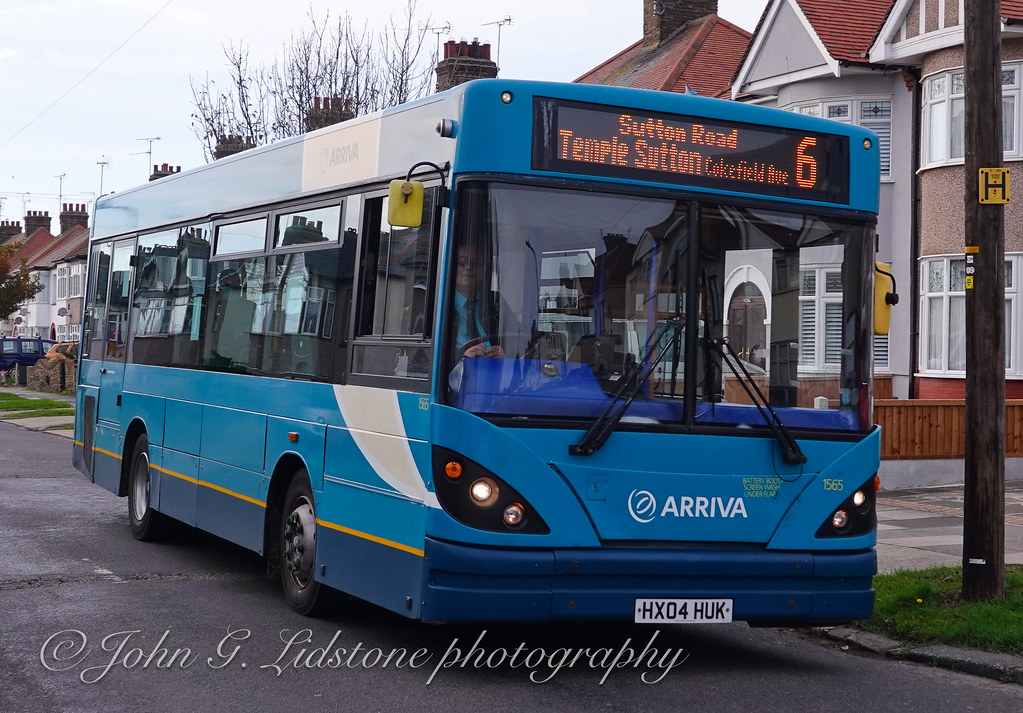This detailed image captures a blue bus parked on the side of a residential street. The bus, marked with "Arriva" and license plate number HX04 HUK, prominently displays an electronic sign reading "Sutton Road, Temple Sutton, Cokefield Avenue, number 6" in orange lights on a black background at the front. In the driver's seat on the right-hand side, a driver donning a light blue shirt and tie can be faintly seen, suggesting the bus is likely in a country where vehicles drive on the left-hand side. The background reveals a row of identical two-story houses, characterized by white facades, slanted brown roofs, and chimneys. Additionally, there is a bus stop with a sign marked "H" nearby. Surrounding the scene are trees, a sidewalk, and grass, reinforcing the residential nature of the area. The bottom left corner of the image is inscribed with the photographer's credit, "John C. Lidstone Photography." The bus appears empty, although it’s difficult to confirm due to window reflections.